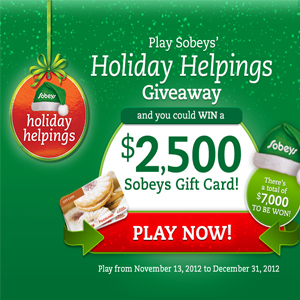The advertisement features a festive theme with a green background that instantly evokes the holiday spirit. On the left side, a red ornament dangles, adding to the seasonal charm. The top part of the ad features the text "Holiday Helpings," adorned with a green Santa hat, enhancing the holiday cheer. Taking center stage, the main text on the right announces "Play Sobeys Holiday Helpings Giveaway" in bold, attractive fonts. Below this, participants are enticed with the opportunity to win a $2500 Sobeys gift card, presented in green text on a white background for emphasis. A prominent red "Play Now" button is positioned prominently, drawing immediate attention with green arrows pointing towards it to guide viewers to take action.

To the right of the "Play Now" button, a small green ball notes that a total of $7000 is up for grabs, further incentivizing participation. At the base of the ad, essential dates are provided, informing participants that the giveaway runs from November 13, 2012, to December 31, 2012. Adding to the visual allure on the left side, several gift cards are displayed, giving a preview of the prizes to be won. The layout and vibrant color scheme effectively capture the holiday theme, while the clear, detailed text ensures that all pertinent information is conveyed to the audience.